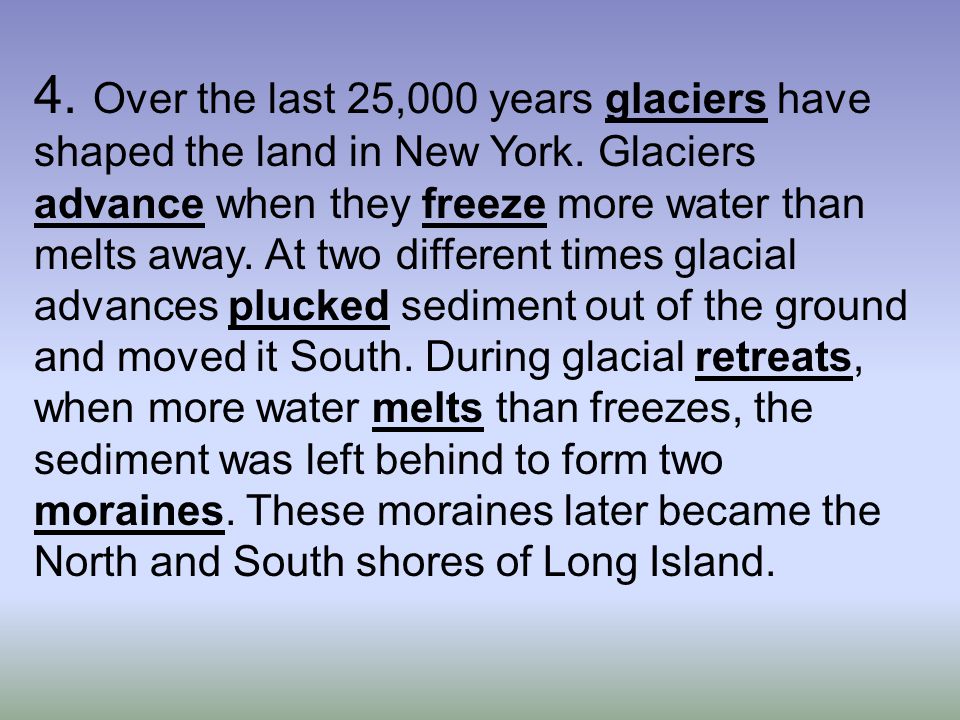The image features primarily text on a gradient background that transitions from medium blue at the top to a grayish-white at the bottom. At the very top, the text begins with "number four." The main body of the text, in black font, states: "Over the last 25,000 years, glaciers have shaped the land in New York. Glaciers advance when they freeze more water than melts away. At two different times, glacial advances plucked sediment out of the ground and moved it south. During glacial retreats, when more water melts than freezes, the sediment was left behind to form two moraines. These moraines later became the north and south shores of Long Island." Key terms such as "Glaciers," "Advance," "Freeze," "Plucked," "Retreats," "Melts," and "Moraines" are underlined and in bold to emphasize important concepts. The top of the background is mainly blue, which gradually fades to white as it reaches the bottom, creating a visually appealing gradient effect.